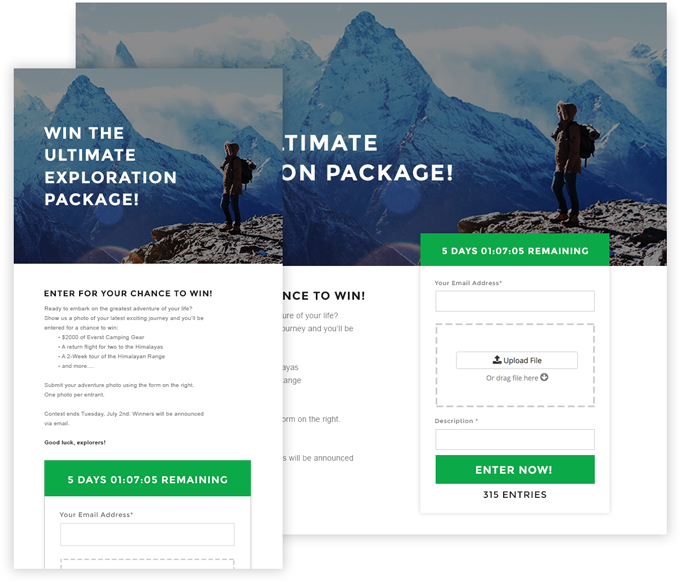This image is a composite screenshot showcasing both a mobile and desktop version of a webpage from an exploration package contest website. At the top of both screenshots is a captivating photograph of a man standing on a mountain peak, gazing over a breathtaking mountain range and an abyss, with snow-capped peaks visible in the background.

In both versions, the phrase "Enter for your chance to win" is prominently displayed. This text is situated beneath the photograph and is followed by some grey text on both the mobile and desktop versions. The mobile version, positioned at the top of the composite image, features a countdown timer at the bottom, indicating "5 days 01:07:05 remaining," emphasizing the contest's limited timeframe.

Below this countdown on the mobile version is a space to enter an email address, an element that is more thoroughly detailed in the desktop version shown underneath. The desktop version also includes a box with a dotted line next to an "Upload File" button for file submissions. Beneath this, there is a text box labeled "Description" and a green "Enter Now" button. Additionally, it notes "315 entries" have already been submitted.

Both versions of the webpage are surrounded by a clean, white background, ensuring that the focus remains on the contest details and the stunning photograph.